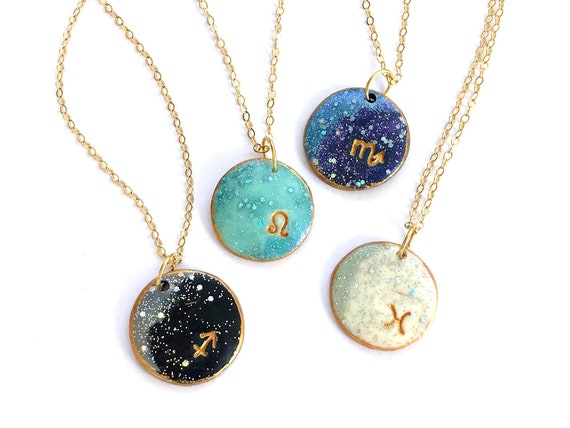This color photograph, oriented in landscape fashion, meticulously showcases four elegant, dainty necklaces with thin gold chains, each adorned with a circular pendant. These pendants, appearing glazed and fired, exhibit a starry background and are distinctively colored in black, teal, navy blue, and green. Each pendant features gold markings or letters in the bottom right corner. The black pendant has a gold arrow pointing to the right, while the teal pendant, representing the Virgo symbol, has a gold engraved symbol. The highest among them, the navy blue pendant, also seems to display the Virgo logo with an arrow pointing upward. Lastly, the green pendant has a symbol resembling an H with curved sides, possibly indicating another horoscope sign. These pendants, arranged side-by-side and appearing to float against a white backdrop, evoke a sense of stylistic photographic representationalism, aimed at detailed product photography.